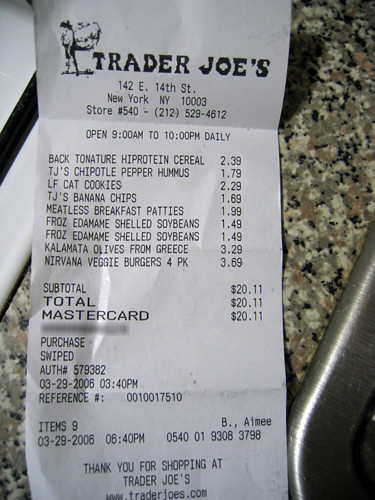The image features a detailed digital photograph taken indoors of a white receipt from Trader Joe's, prominently placed near the center of a shiny, marble-like countertop. The marble surface is a speckled mix of white, cream, gray, and black, contributing to a polished appearance. In the bottom right corner of the image, there's a silver, possibly stainless steel, object that could be part of a sink.

The receipt itself, written in black text on white paper, shows the Trader Joe's logo featuring a person carrying a large bag. It lists the store's location at 142 East 14th Street, New York, NY 10003, with the store number 540. The receipt details various purchased items, with a subtotal and total amount of $20.11, noted to be paid via MasterCard. At the bottom of the receipt, additional text includes a thank you message and the store's website, www.traderjoes.com. Some parts of the receipt appear blurred, likely to obscure sensitive information.